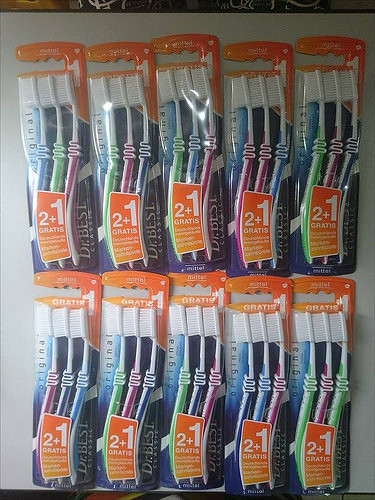The image features a display of ten vertically standing toothbrush packages, each containing three toothbrushes. The packages are organized into two rows with five packages per row. Each package has an orange top with a dark-colored body. Every package prominently displays an orange label that reads "2+1 GRATIS" in white text, indicating a buy two, get one free offer. The toothbrush handles come in blue, green, and purple, with distinct squiggly lines near the top of each handle. The bristles on all toothbrushes are white. The background of the display is a light gray color.